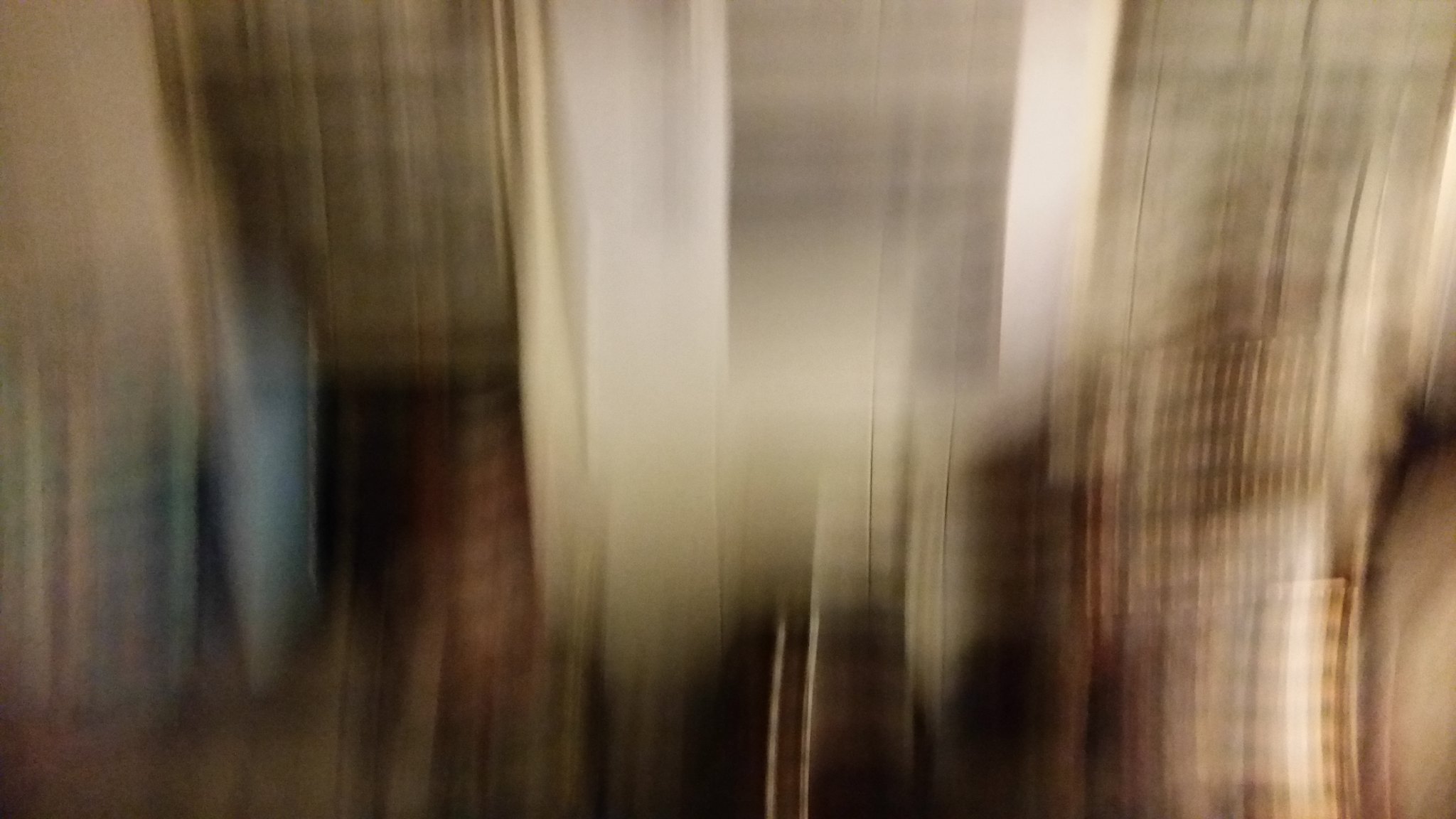In this extremely blurry and stretched image, it is challenging to discern specific details due to significant blurring, likely from camera movement. The image appears to depict an interior scene with bright colors. On the left side, there is a stretched blue area, while on the right, there is a similarly stretched white and tan section. The center prominently features what looks like a window or a doorway, surrounded by a white frame, which could also be part of a white wall. The bottom right showcases a boxy outline with a brown border and stripes, which might be a throw pillow or a frame, though it is indistinguishable due to the distortion. The overall scene is well-lit, suggesting an indoor environment.